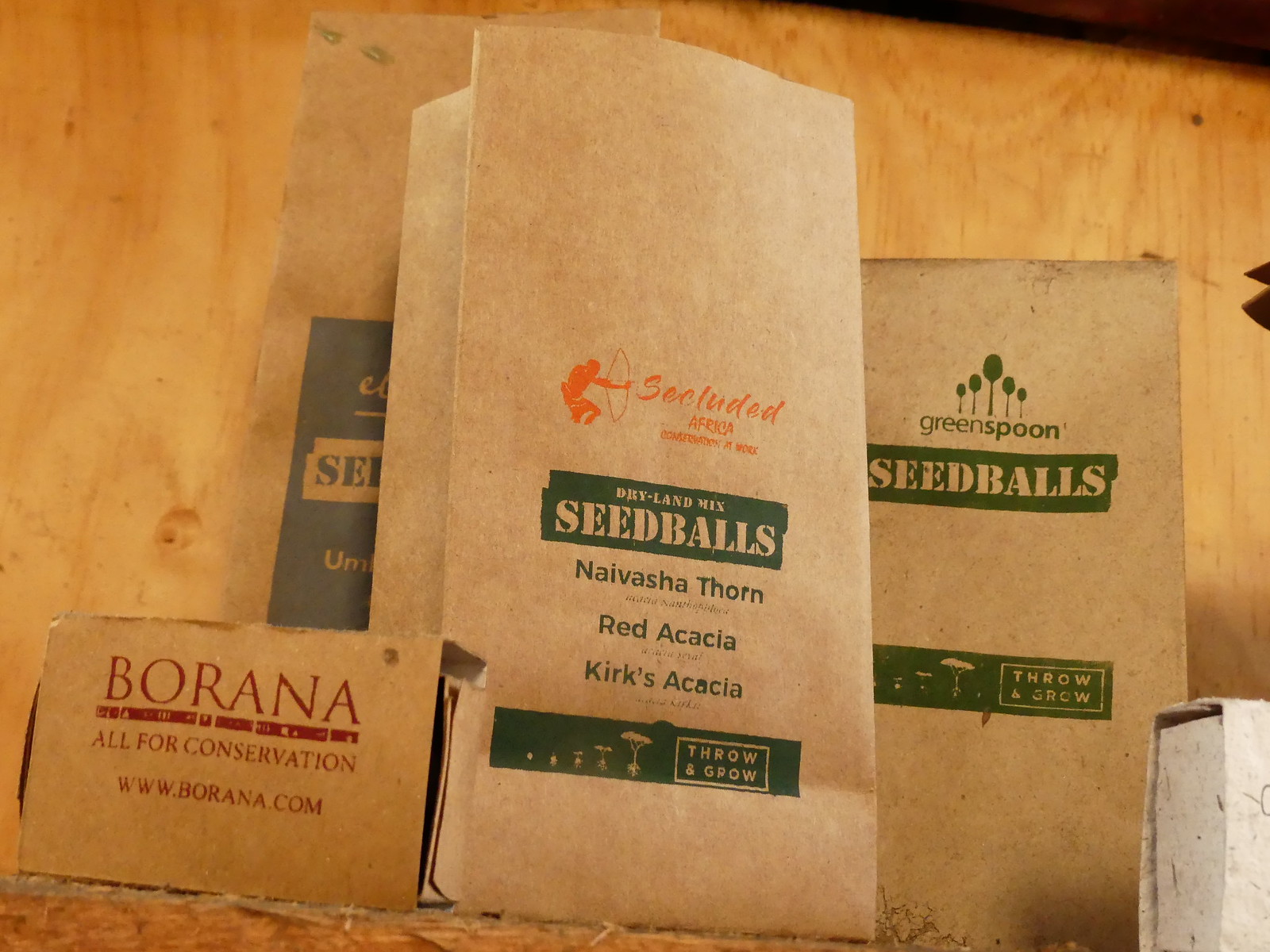This indoor photograph showcases a rustic wooden table adorned with an assortment of eco-friendly packaging. Central to the composition is a brown paper bag labeled "Secluded African Commentary at work, Dryland Mix Seed Balls: Naivasha Thorn, Red Acai, Kirk's Acai. Throw and Grow," with text in green. To its right is another brown paper bag marked "Green Spoon Seed Balls Throw and Grow," suggestive of being from the same company. On the left, another brown bag features "Seed Balls" written in blue, consistent with the natural theme. In the bottom left corner, a small rectangular brown cardboard box displays the message "Borana, all for conservation, www.borana.com" in red lettering. The backdrop consists of an unfinished panel of light-colored, yellowish plywood, enhancing the rustic and eco-conscious ambiance of the photograph.